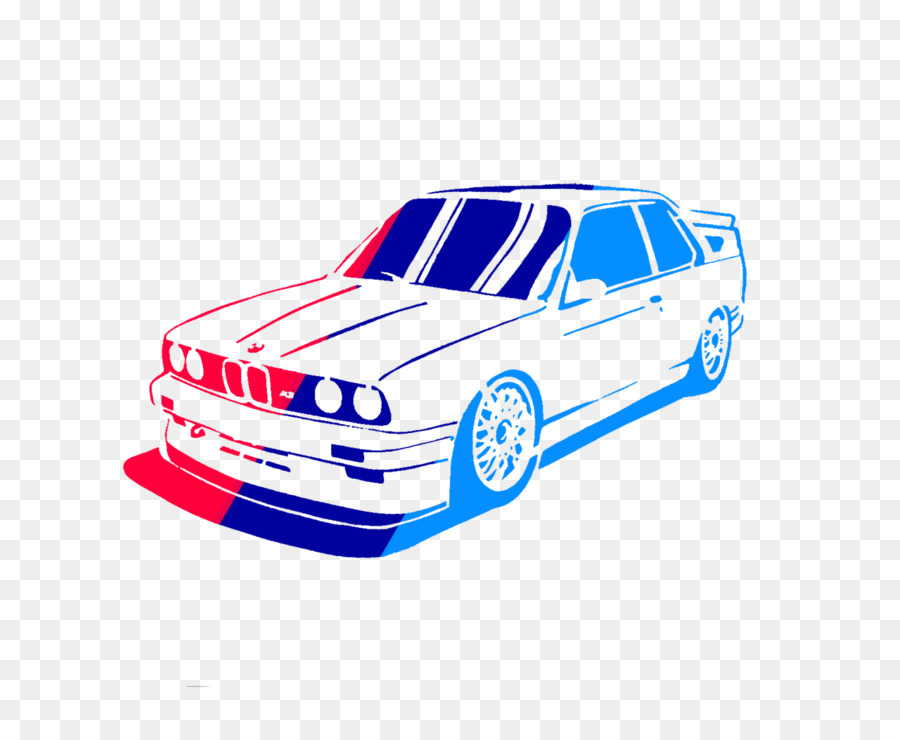The image depicts a digital art drawing of an older, boxy BMW coupe, possibly from the 80s or 90s, set against a gray and white checkerboard background commonly associated with Photoshop's transparency pattern. The car features a prominent, flared bumper reminiscent of rally cars, dual circular headlights on each side, and a two-piece rectangular grille with a likely BMW emblem on the hood. It has sporty spoked rims and a rear spoiler. The car is adorned with a racing stripe that runs from front to back, composed of three colors: red, dark blue, and light blue. These colors are also visible across various parts of the car, including the windshield and other windows, which are tinted in shades of blue. Additionally, the car's underside and wheels reflect a combination of light blue, dark blue, and red hues, contributing to a shadowed effect beneath the vehicle.